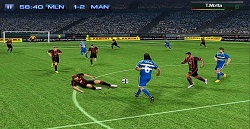The image appears to be a screenshot from a soccer video game, likely from the FIFA series. The main focus is on a green soccer field with low-resolution graphics showcasing digital players in action. At the top of the screen, there is a scoreboard displaying a score of 56 to 40. Beneath the scores, it reads "Men 1 - 2 Man," likely indicating a team matchup or game status. Additional text is present in the top right corner, but it's too small to decipher. In the background, large bleachers filled with a virtual audience intently watching the game can be seen, adding to the immersive atmosphere. One team is dressed in blue uniforms, while their opponents are clad in dark red. The overall visual quality suggests an older or lower-quality version of the game.